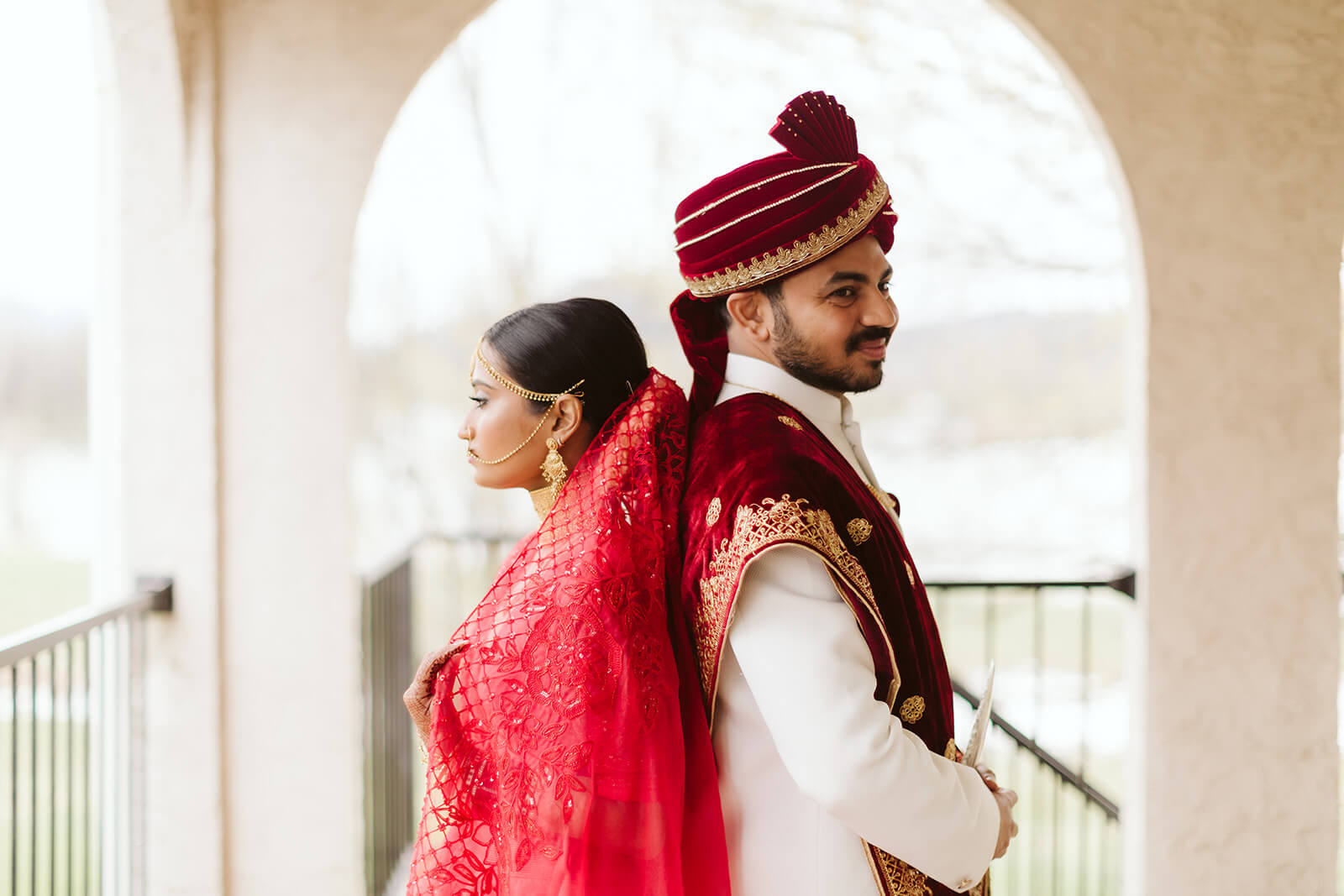This is a photograph of an Indian couple standing back-to-back in an ornate archway. The woman, on the left, is adorned in a beautifully embroidered red dress and a translucent red shawl with a floral design. Her traditional gold jewelry includes an intricate forehead piece that connects to her left ear and mouth, along with large golden earrings. She gazes softly to the left. The man, on the right, wears a white long-sleeve coat paired with a red velvet sash adorned with gold ornaments draped over his right shoulder. He completes his regal look with a maroon velvet turban featuring elaborate designs. Smiling, he looks to the right. Behind them, the white arch with black railings and a blurry background of tree branches adds a timeless, cultural elegance to the scene.